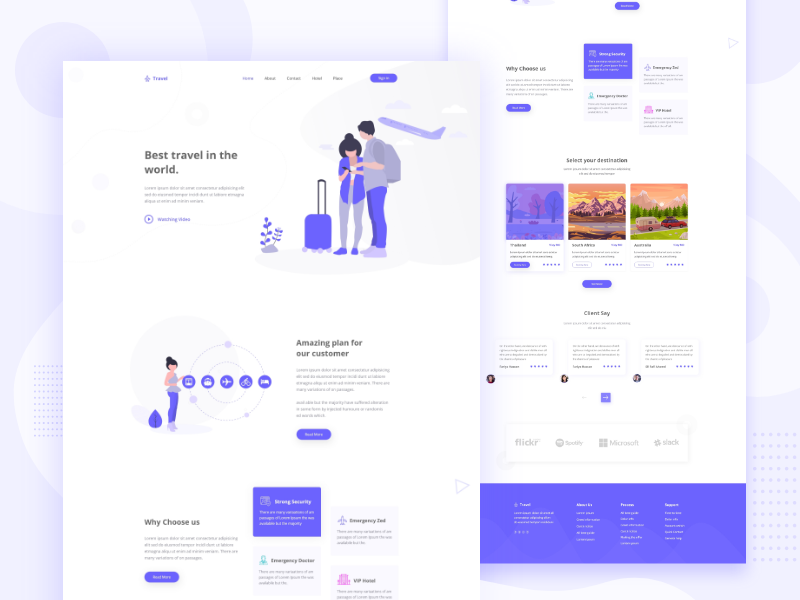The image shows a website page that caters to travel services, featuring two sections side by side. The left section is positioned slightly lower than the right section. The right section prominently displays the headline, "Best Travel in the World." Adjacent to it on the left is a simplified illustration of a man and woman standing side by side with a plane in the background. The figures, depicted without facial features and minimal dark outlines, are shown holding a piece of luggage and looking at their phone.

Beneath the illustration, the text reads, "Amazing Plan for Our Customer" followed by the headline, "Why Choose Us" on both sections. The right section further elaborates on the reasons to choose their service through a series of three small boxes listed under "Select Your Destination." At the bottom of the right section, there is another set of three boxes under the headline, "Clients Same," which includes images of individuals on either side. However, all other text within the section is too blurry to read.